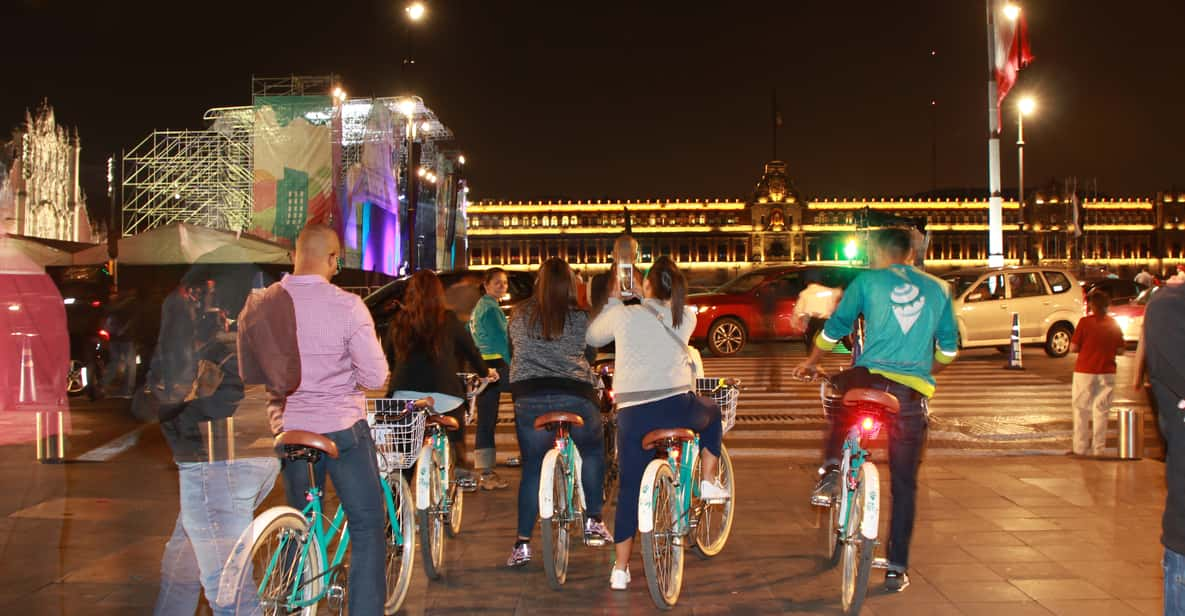The photograph depicts a bustling nighttime scene in an urban environment, characterized by a black sky tinged with brown hues. Central to the image are numerous people riding distinctive green-framed bicycles equipped with brown seats and white tire protectors. A notable rider in a purple shirt commands attention amidst the activity. The scene is further populated with various cars, including red and silver ones, navigating the streets. A crosswalk is visible where pedestrians, such as a woman in a red shirt and white pants, are standing on the curb. The urban backdrop features buildings adorned with yellow lights, emphasizing the lively city atmosphere. Overhead, a bright golden lamp post light illuminates part of the scene, and a flag with a white top and red bottom is attached to the pole. The entire composition underscores the dynamic interplay between cyclists, pedestrians, and vehicles in a vibrant cityscape.